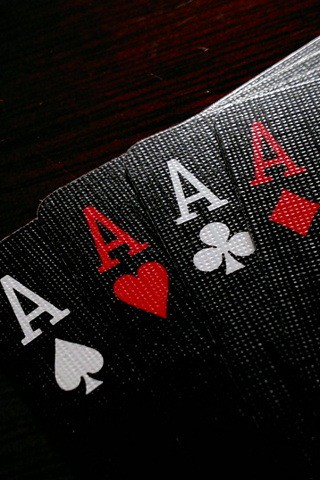The image features a background that transitions from a blackish hue on the left to a dark brown, wood-like texture on the right. The gradient provides a rich, rustic contrast to the foreground. In the foreground, there are four playing cards arranged from left to right, each predominantly black with white vertical stripes near the top that fade into pure black towards the bottom.

Starting from the left, the first card displays a white 'A' and a spade symbol. The next card, positioned slightly higher and to the right, shows a red 'A' with a heart symbol. Following this is another card, slightly above and to the right, featuring a white 'A' and a club symbol. The final card, also to the right, showcases a red 'A' with a diamond symbol in red.

These cards become increasingly challenging to discern as they progress to the right due to the white lines blending into the lighter background. The last card, the ace of diamonds, is particularly difficult to make out.